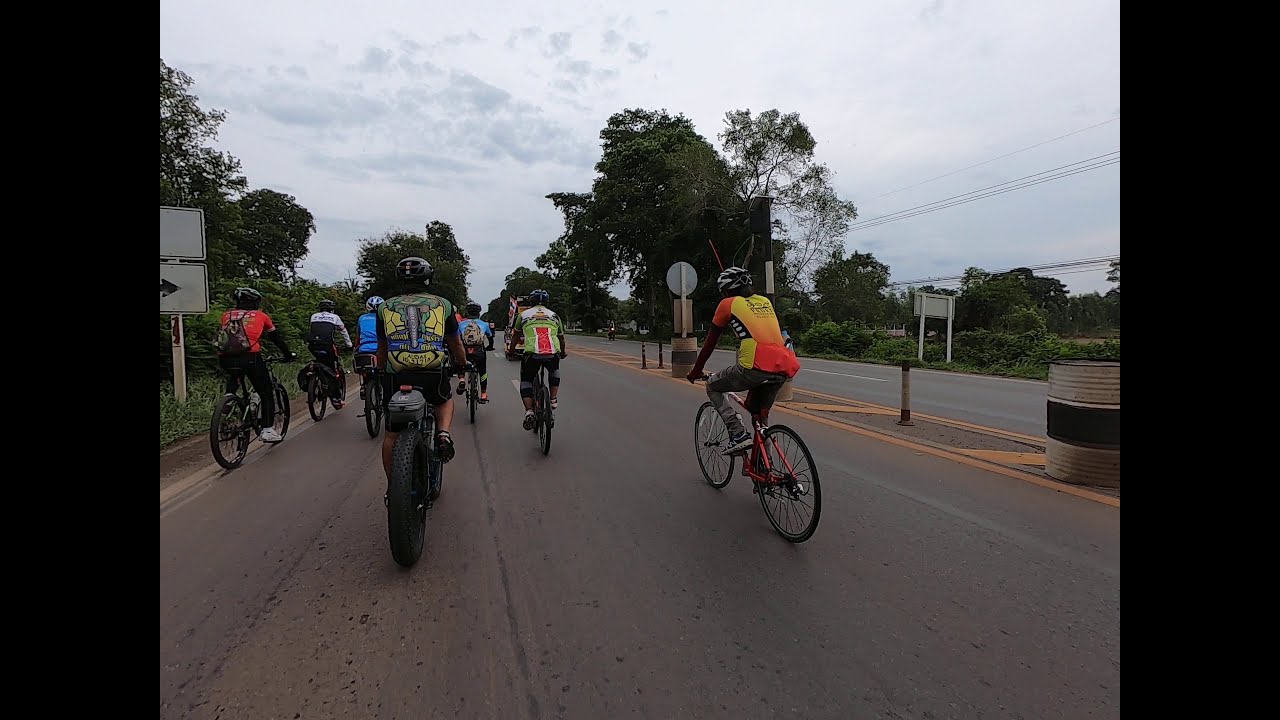The image captures the dynamic scene of a casual bike ride involving eight individuals, adorned in bright, multi-colored cycling outfits including tight shirts, shorts, and black helmets. They ride on the left side of a two-lane asphalt street, with the right lane open and devoid of traffic. A yellow-outlined median, which houses several black and white multicolored barrels, separates the lanes. The landscape orientation photograph, possibly a freeze-frame from a GoPro video taken from a helmet-mounted camera, provides a view from behind the cyclists as they pedal into the distance. The left and right sides of the street are lined with green grass, shrubs, tall trees, and telephone wires visible on the right. White signs can be seen erected on both sides of the road, facing away. The sky is a light blue, dotted with clouds, adding to the daytime ambiance. Each bicycle enthusiast is riding a different type, including notable appearances of a fat tire bike and a skinny tire bike, contributing to the diversity of the scene.